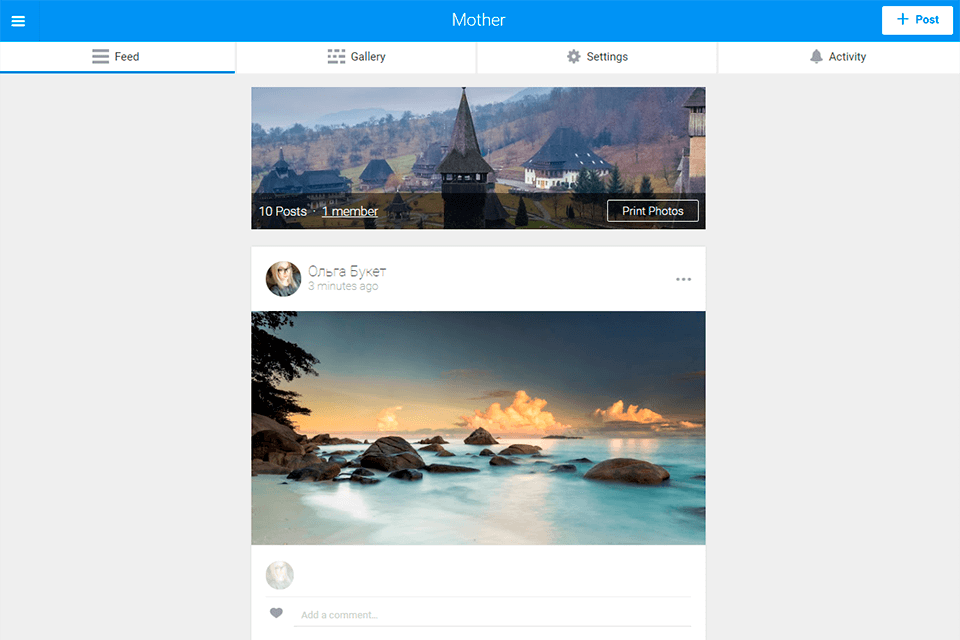At the top of the image, there is a blue rectangular bar featuring a hamburger menu on the left. Below this, a feed begins with a post from a mother. The interface continues to display various sections such as a gallery, settings, and activity.

The central image showcases a serene landscape with buildings, their rooftops visible amidst scattered fields and trees, and a prominent temple structure. In the foreground, there’s another blue rectangular section with the text "Print Photos."

Further down, there's a picture of a person wearing glasses, with their name stylishly written in acrylic font. This post was made three minutes ago, indicated by the text "three minutes ago..."

Towards the bottom of the page, the image displays a dark sky with dazzling yellow clouds. Below this, serene blue waters with smooth textures flow around visible rocks, and a tree is positioned to the left of the image.

At the very bottom, a red heart icon is present, seemingly indicating a like or love reaction, set against a grey background. The caption concludes with a cheerful sign-off: "Thanks for watching!"